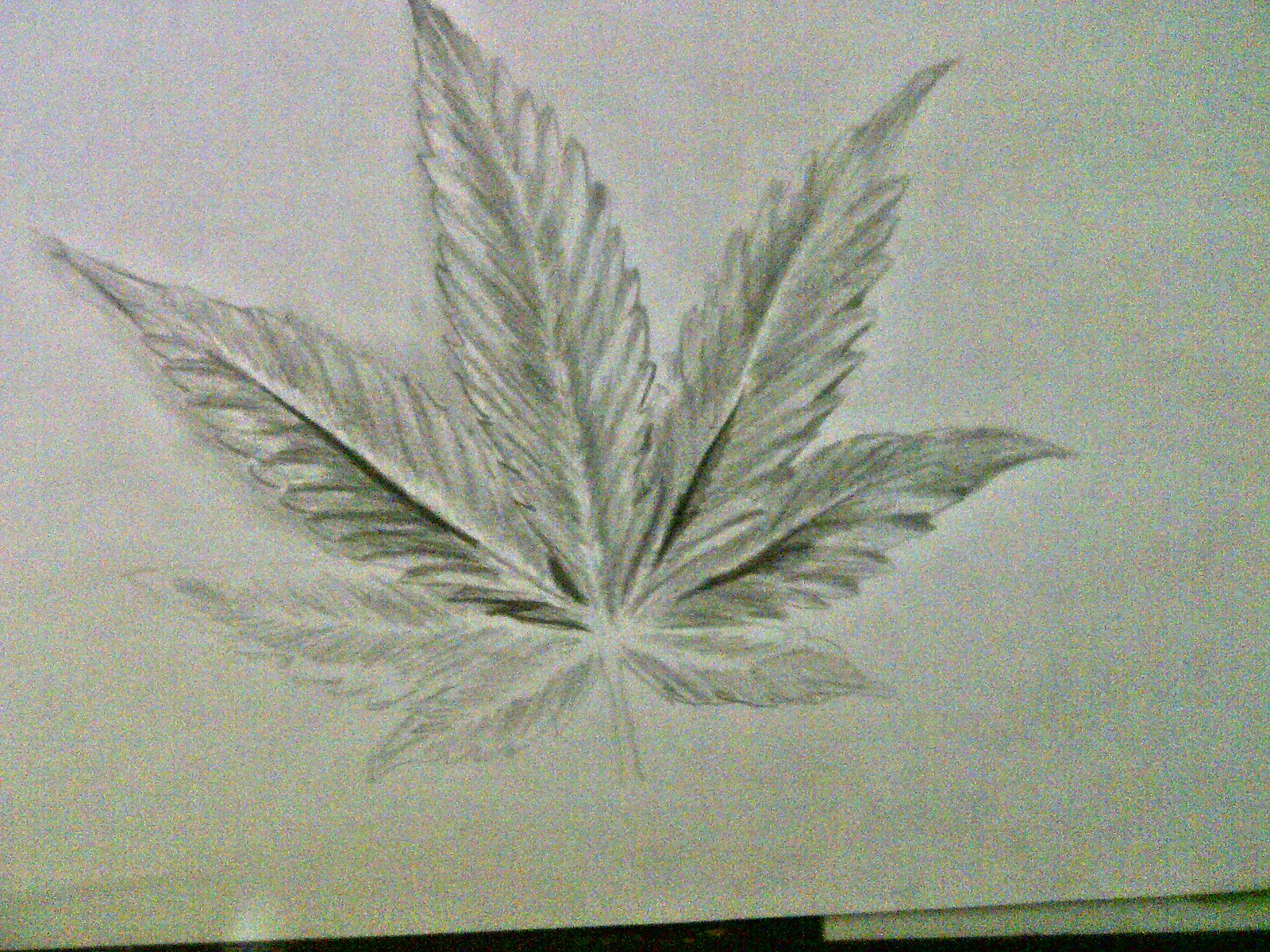The image captures a slightly out-of-focus photograph of a pencil sketch of a distinctive pointy leaf, positioned against a white background with faint light green shading. The sketch is likely of a marijuana leaf, characterized by its star-shaped pattern and multiple jagged edges. The leaf consists of seven distinct lobes with varying degrees of shading, and a visible stem extends upward from the bottom center of the drawing. The lower edges of the leaves appear slightly blurred due to the photo's focus, yet the texture and details of the sketch are evident. The presence of the paper's edge at the bottom of the image and another sheet behind it confirms it's a photo of the sketch. Each lobe is meticulously drawn, with the central ones stretching out vertically and the side lobes extending outwards and downwards from the central stem, collectively forming a recognizable and detailed representation of the leaf.